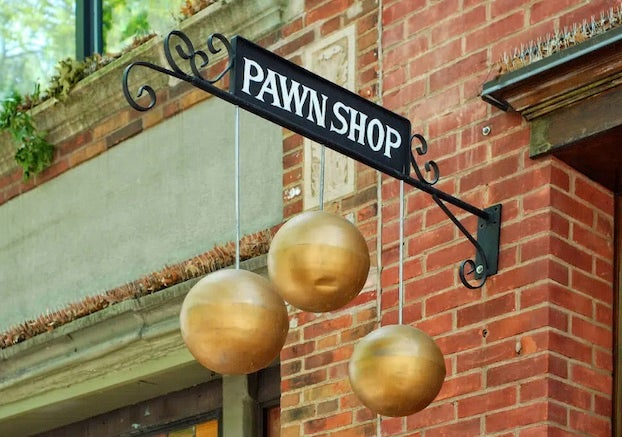The photograph showcases the exterior sign of a pawn shop, captured in landscape mode and in color. The sign, a wrought iron masterpiece, extends perpendicularly from a stately red brick building, creating an elegant and upscale appearance. Large white letters spelling out "Pawn Shop" stand starkly against a black background, drawing immediate attention. Beneath the sign, three golden orbs hang decoratively, adding a touch of classic charm. The building's architecture is meticulously detailed, featuring different borders and a weathered brass lintel above the entry door. Adjacent to the pawn shop, a gray cement facade edged with red brick adds contrast. The scene is further enriched by the presence of some leaves sprouting from the gutters and a hint of foliage in the upper left-hand corner, evoking a sense of nature amidst the urban setting.